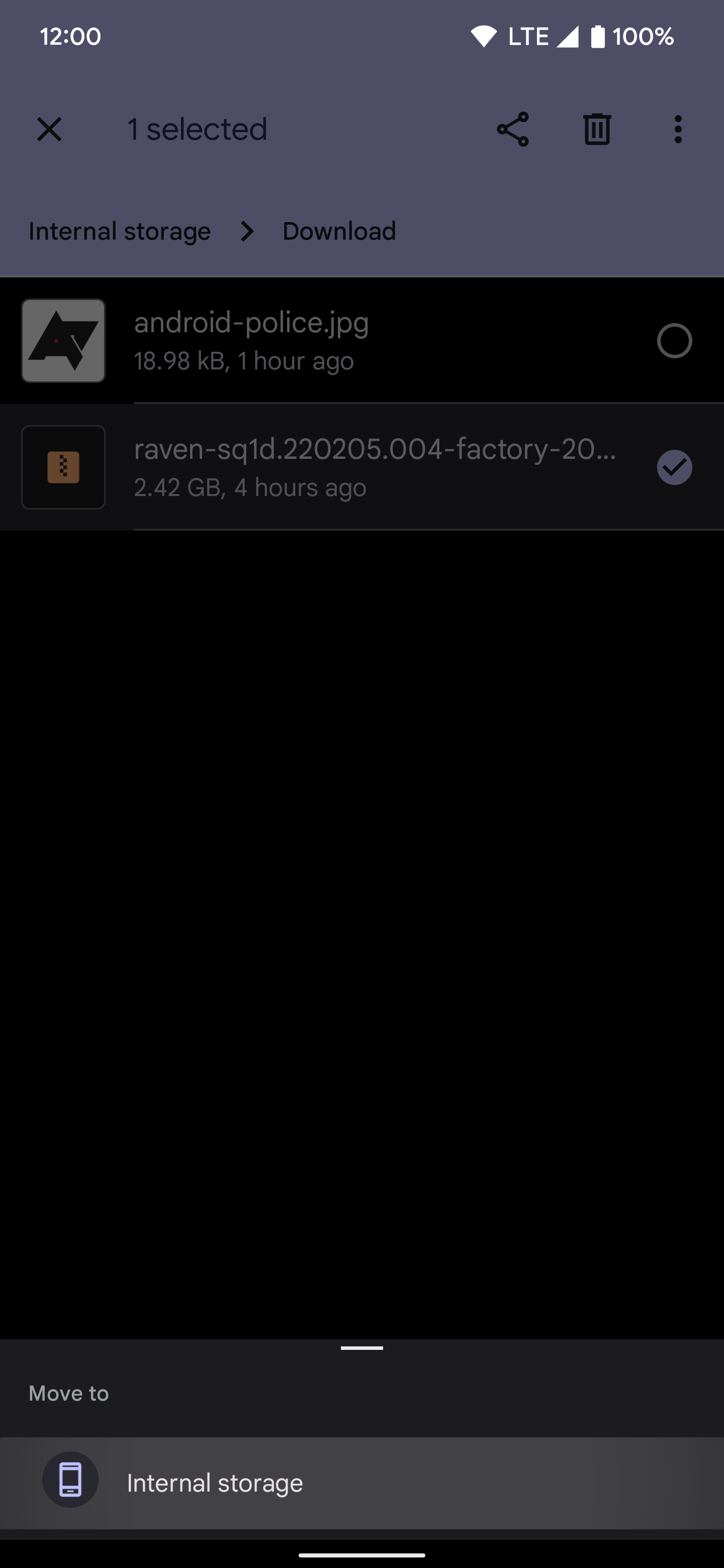A screenshot captured from a smartphone screen shows several elements in a detailed view. At the top, a dark grayish background banner displays the time "12:00" in white letters, alongside indicators for LTE signal strength and a fully charged battery, both in white. 

Within this banner, black lettering specifies “1 selected” to the left of an "X" icon, while the right side features a set of interconnected three circles forming a triangle, adjacent to a trash can icon and three vertical dots. 

Below this section, "Internal storage" is labeled in black letters, followed by a greater-than symbol (>), leading into a section labeled "Download."

The main background of the screen is black, showing two horizontally listed items. The first item features a white icon resembling the letter "A" with a triangle in black, labeled "android-police.jpg" in white text. Below this label, it indicates a file size of "18.98 kilobytes" and a timestamp of "one hour ago." To the far right of this item is an open circle.

The second item displays an icon described as a black circle enclosing an orange square with a black squiggle in the middle. The text next to this icon reads "raven-sq1d.220205.004-factory-20..." showing a file size of "2.4 gigabytes" and a timestamp of "four hours ago." To the right of this entry, a gray-filled circle with a black check mark is visible.

At the bottom, a slightly lighter black banner reads "Move to" in light gray letters. Below this banner, a lighter gray band at the very bottom of the screen shows a small phone icon with the white text "Internal storage."